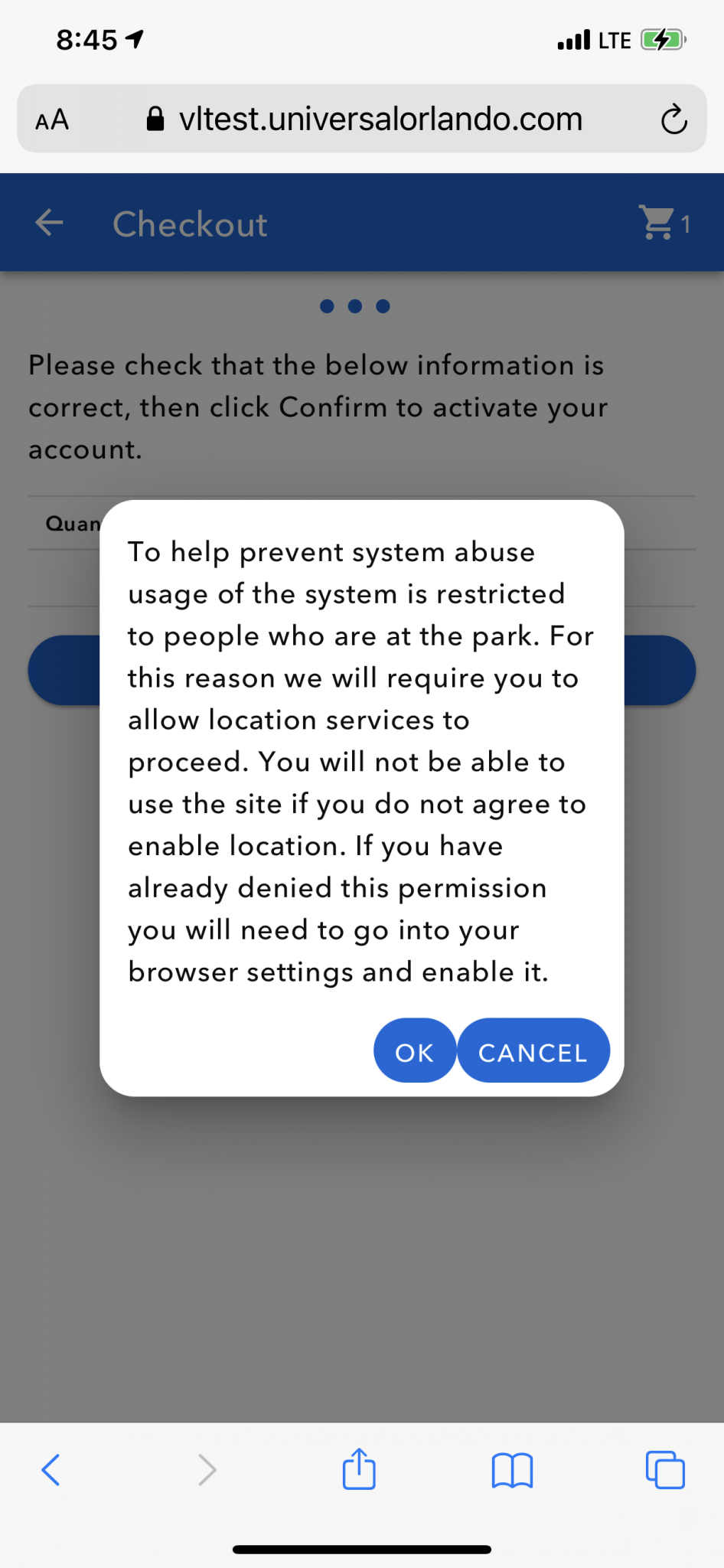This composite image consists of two panels side by side. 

**Left Panel:**
- The panel on the left is a screenshot from a cell phone. 
- At the top edge of the screen, typical status indicators are visible: the time “8:45,” the "LTE" connection type, a cell signal indicator, and the battery level.
- Just below these indicators is a darker gray search or address bar displaying the URL "vltest.universalorlando.com" with a padlock symbol indicating a secure connection.
- The main focus of this panel is a pop-up message that appears under a blue banner which likely signifies the checkout section of a website. 
- The pop-up has a warning in white text on a blue background, stating: “To help prevent system abuse, usage of the system is restricted to people who are on or at the park. For this reason, we will require you to allow location services to proceed. You will not be able to use this site if you do not agree to enable location. If you have already denied this permission, you will need to go into your browser settings and enable it.”
- The message is followed by "OK" and "Cancel" buttons, contained within blue circles, indicating actionable responses.

**Right Panel:**
- The panel on the right has a yellow background and features a large square.
- Inside the square there is text that prompts the viewer to think critically about the image: "Think about what the image is at first glance. What are the objects and their contents? What does the text say? What are the positions of the objects? What subtle details are noticeable? What is the background and what is the style and color?"
- This text encourages an analytical viewing of the image, focusing on details and contextual clues.

The contrasting designs and purposes of the left and right panels invite a viewer to consider not just the primary information provided but also the visual composition and contextual elements of the entire image.